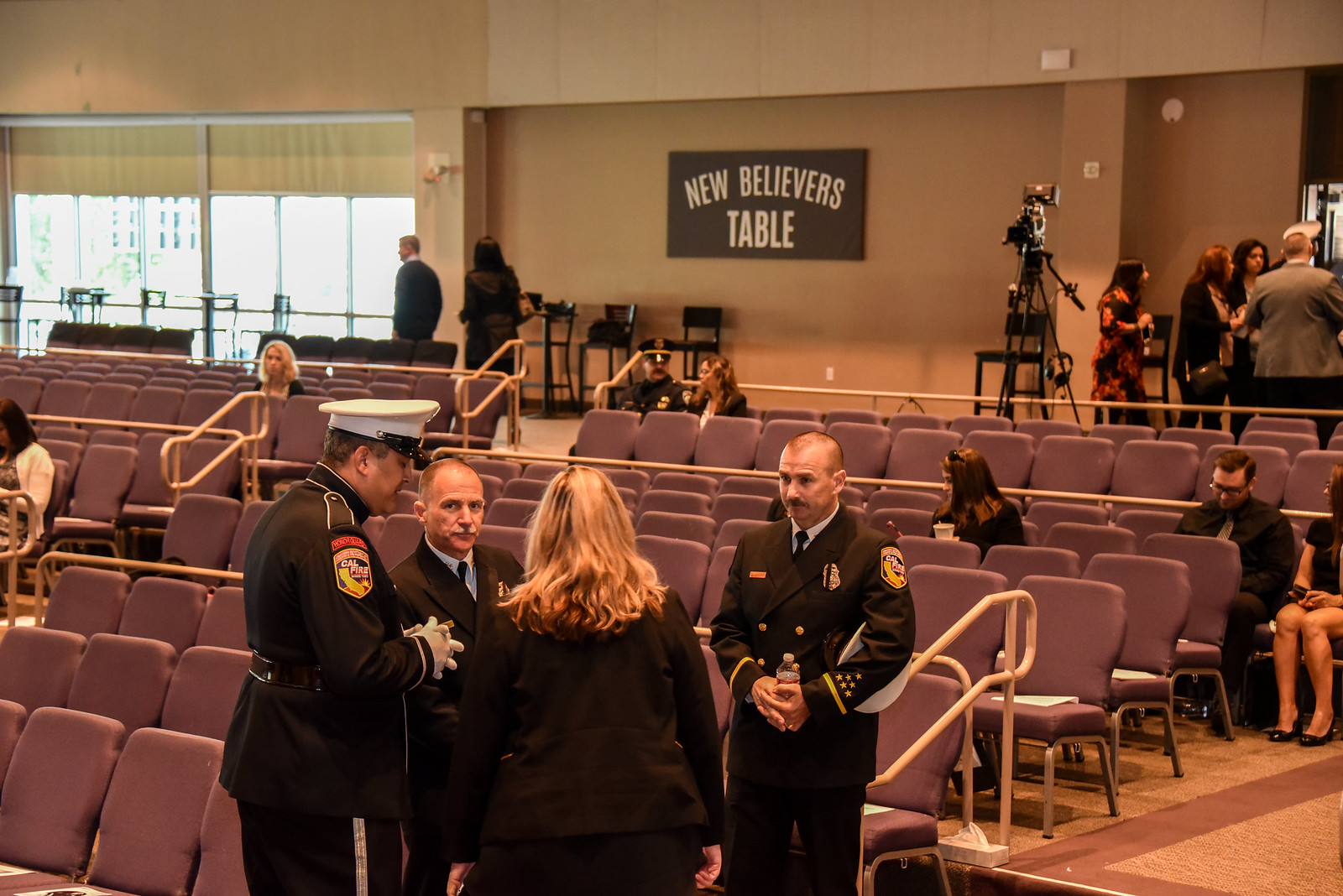The photograph captures an indoor scene within a large church or auditorium, oriented towards the back of the room. In the foreground, four individuals dressed in black uniforms with "CAL FIRE" patches stand conversing. Two of them appear to be firefighters, while the exact roles of the others are ambiguous due to the lack of visible gold badges. To the left, one firefighter is distinguishable by a white and red cap. Directly behind them, an evenly spaced arrangement of purple chairs populates the area, with a few individuals seated or standing nearby. Above this gathering, a prominent black sign with white text reads "New Believers Table" affixed to the back wall. To the right of the sign, a camera mounted on a large stand is manned by a few people standing beside it. Further left, near a set of windows allowing natural light to penetrate the space, additional attendees are visible, adding to the sense of a post-event atmosphere. The well-lit room, filled with scattered groups engaged in conversation, suggests the conclusion of a service or meeting.